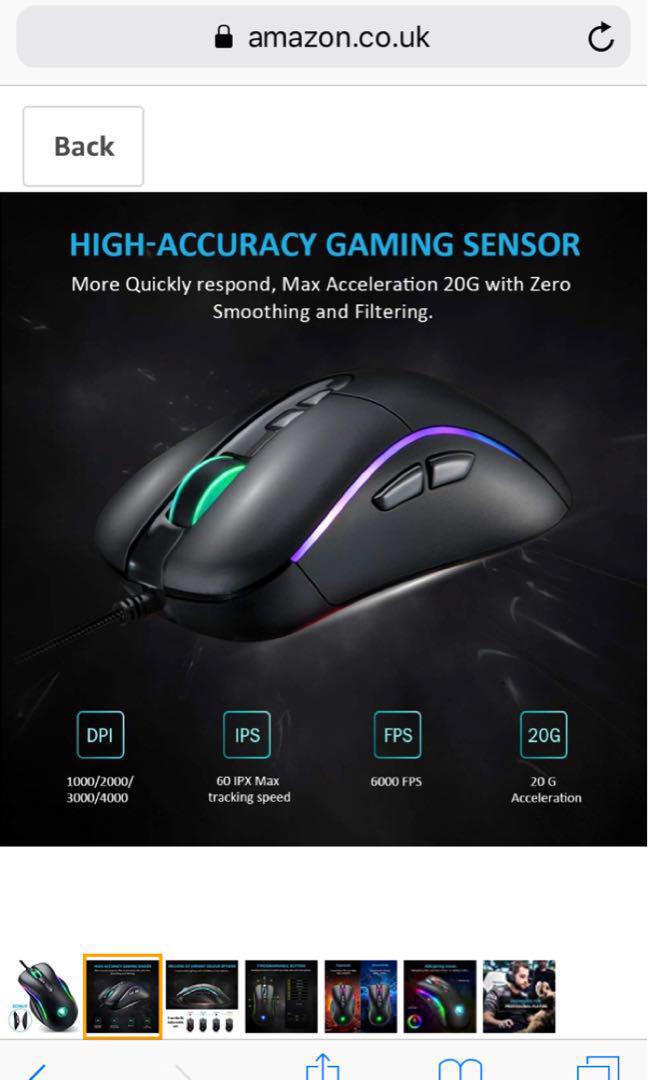The image appears to be an advertisement for a high-precision gaming mouse displayed on the Amazon.co.uk website. The top of the page features the Amazon.co.uk logo and a refresh icon to its right. Below that, a back button is present, though it does not seem to be selected. Adjacent to it is a black square that showcases the product.

The focal point of the image is the gaming mouse, accompanied by the headline "High Accuracy Gaming Sensor" in blue text. Below this, in white text, it states, "More Quickly Respond Max Acceleration 20G with Zero Smoothing and Filtering." The mouse itself is sleek and black.

Beneath the mouse's image, there are four rounded icons indicating key features: DPI, IPS, FPS, and 20G. Additionally, there are seven smaller squares likely representing alternative views or options for the product. One of these shows the mouse on a white background tilted at an angle, similar to the main display. Several other views of the mouse are also depicted, each providing different perspectives. The final image in this row appears to show at least one man, potentially in a conversational setting though the details are unclear.